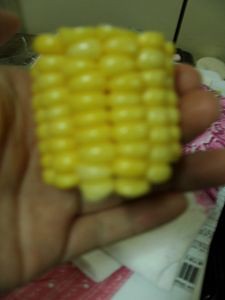In this color photograph, a small, baby-sized piece of corn on the cob is held in the open palm of a Caucasian person's hand, with their fingers slightly closed around it. The vibrant golden yellow kernels, fully formed and healthy, are in sharp focus despite the slightly blurry details around the edges. The foregrounded hand, including visible lines and finger tips but not the thumb, holds the corn up to the camera, making it the main focus of the image. Behind the hand, a layered arrangement of papers is visible: a white and patterned pink paper plate on top, underpinned by white papers with indistinct writing and a barcode or ISBN label visible. A pinkish table surfaces underneath these items, with additional background details including a black item with a long cord and possibly a white bowl. It all comes together to create a vivid and textured close-up shot emphasizing the corn and the hand holding it.